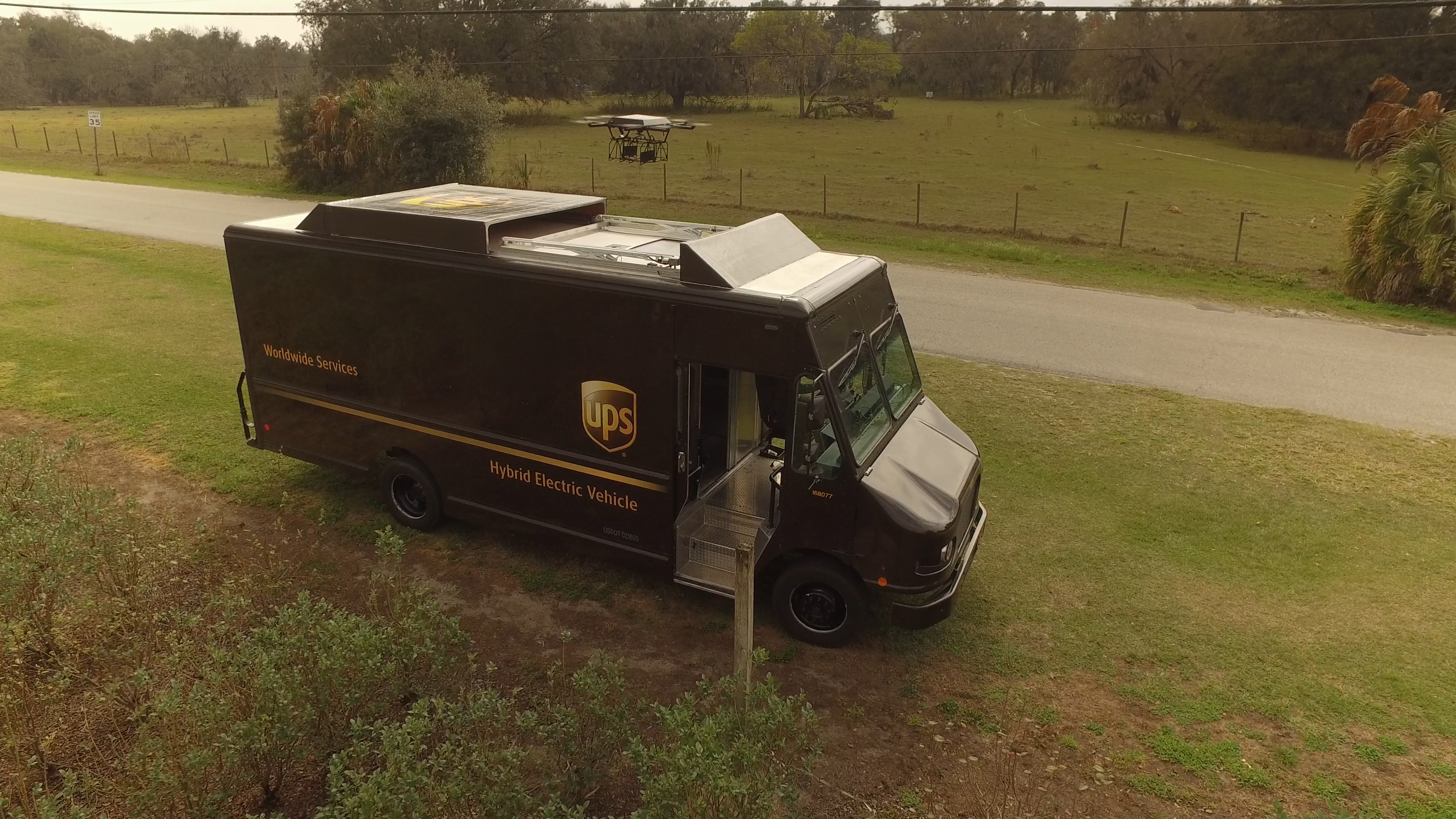The image depicts a dark brown UPS delivery truck with the classic gold UPS logo and text indicating "Worldwide Services" and "Hybrid Electric Vehicle." The truck, with its rectangular shape and open door, is parked in a grassy field that features patches of dirt. Atop the truck, there appear to be solar panels or a drone, suggesting sustainable technology. The background reveals an asphalt road with a 35 MPH speed limit sign, beyond which stretches another grassy field dotted with trees, bushes, and a wooden post. Overhead, there's a visible power line. The shot, likely taken by a drone given its elevated angle, captures the scene in daytime lighting.